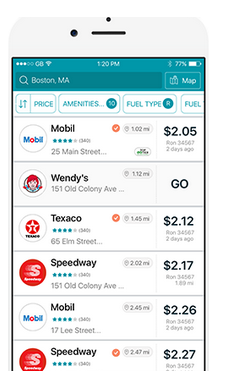The image displays a search interface specific to finding fuel stations in Boston, Massachusetts. At the top, there's a search bar accompanied by a magnifying glass icon with the text "Boston, Massachusetts". To the right of the search bar, there's a "Map" button.

Below the search bar, there are several filter options: an up-and-down arrow labeled "Price", a box labeled "Amenities", and another box labeled "Fuel Type". Underneath these filters, there's a section labeled "Set Mobile" with a mobile icon.

The first listing shows a rating of four out of five stars and details for a location at 25 Main Street, which is 1.02 miles away and offers fuel at $2.05, updated two days ago. Adjacent is the Wendy's logo, indicating an affiliated Wendy's at 151 Old Colony Avenue, 1.12 miles away. The right column notes this location with the label "Geo".

The second listing is for Texaco, showing their icon on the left, four out of five stars, located at 65 Elm Street, 1.45 miles away, with fuel priced at $2.12, last updated two days ago.

The final listing is for Speedway, marked with their icon, located at 151 Old Colony Avenue, 2.02 miles away, with a fuel price of $2.17.